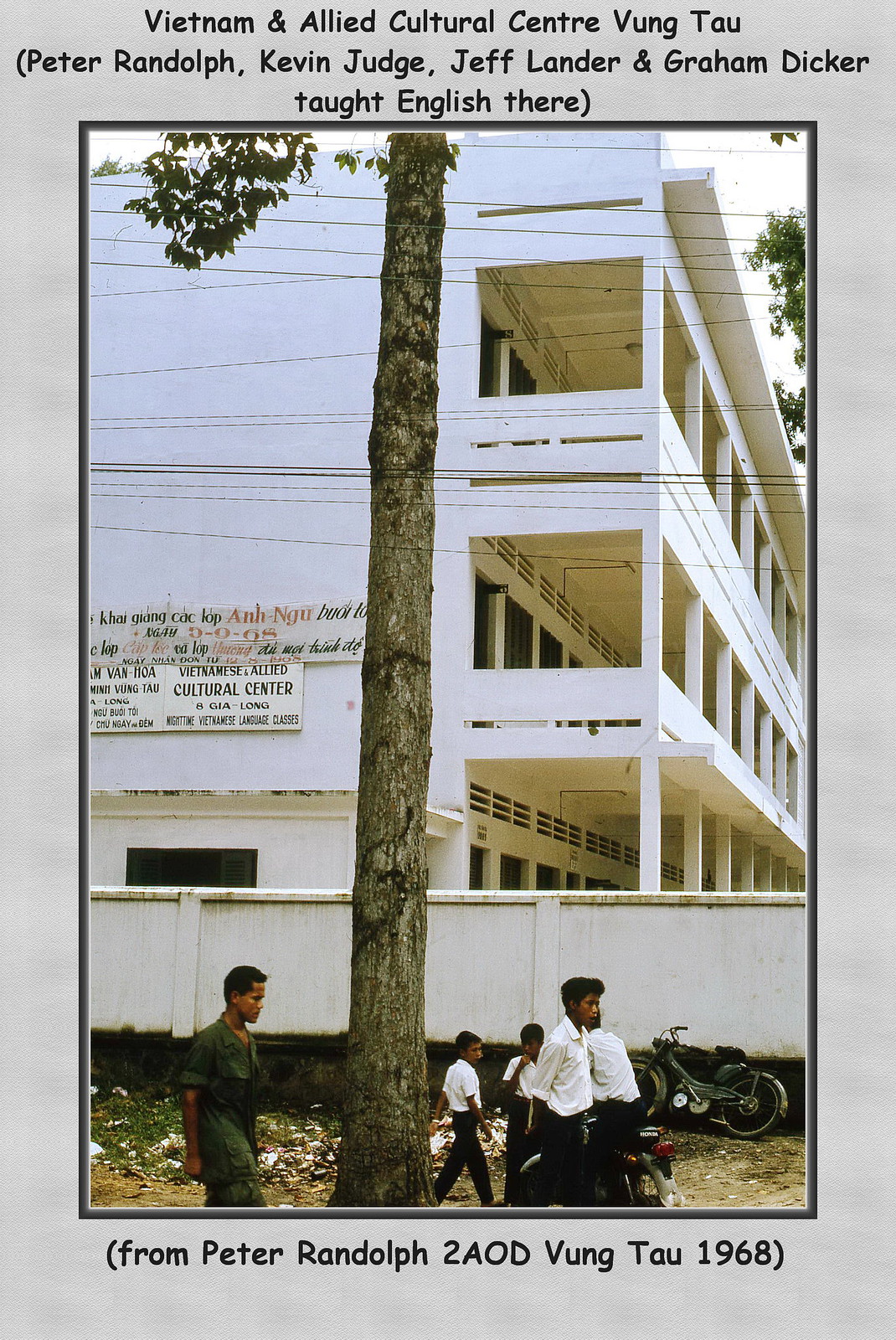The postcard, presented in portrait form, features a vintage color photograph from 1968 inset into a light gray background with a gray outline. At the top, black text reads, "Vietnam and Allied Cultural Center, Vung Tau (Peter Randolph, Kevin Judge, Jeff Lander, and Graham Dicker taught English there)." Below, another caption in black type states, "From Peter Randolph, 2AOD, Vung Tau, 1968."

The photograph showcases a three-story white building identified as the Vietnamese Allied Cultural Center, indicated by signage on the building's top left on the second floor. In the foreground, several Asian students in white shirts and black pants stand by a tree, accompanied by a soldier in a green uniform patrolling the perimeter. A bicycle leans against a wooden fence near the building. The image, captured during the daytime, combines elements of vintage color photography with precise typography in a graphic design style.